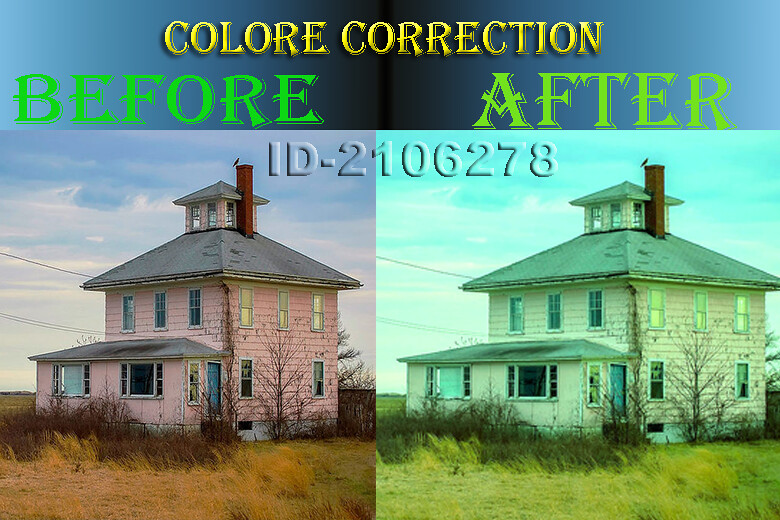The image features a color-modified example of a house, presented as a before-and-after comparison. At the top of the image, set against a blue gradient background, the words "COLOR CORRECTION" are prominently displayed in yellow letters, with "color" uniquely spelled as "C-O-L-O-R-E." Below this title, the left side is labeled "before" in green text, while the right side is labeled "after," also in green. Directly beneath these labels, the same house is shown in two states. On the left side, the house appears weather-beaten with pink panels, gray shingles, and a brick chimney topped by a bird. Surrounding the house are dead trees, dead grass, and dead brush. The windows, framed in white, display peeling pink paint. In contrast, the right side of the image presents the house color-corrected to a light yellow hue. The sky is depicted in a lighter blue tone, and the grass and vegetation in front of the house appear brighter and healthier, with a yellowish tint. The only elements that remain unchanged are the chimney and the bird. A sequence of letters and numbers, "I-V-2106278," blends into the background between the two pictures, yet is visible due to its shadowed effect.